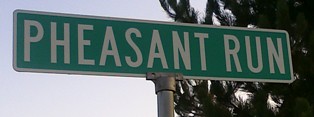The image features a detailed close-up of a street sign positioned against a pale blue sky with a slight whitish hue. Only the top portion of the metal pole is visible, showcasing the last few inches before meeting the elongated, horizontal sign. The sign itself is green with a white border, displaying the text "Pheasant Run" in bold white letters. To the right of the sign, a tall pine tree stands, its branches allowing glimpses of the serene sky beyond.